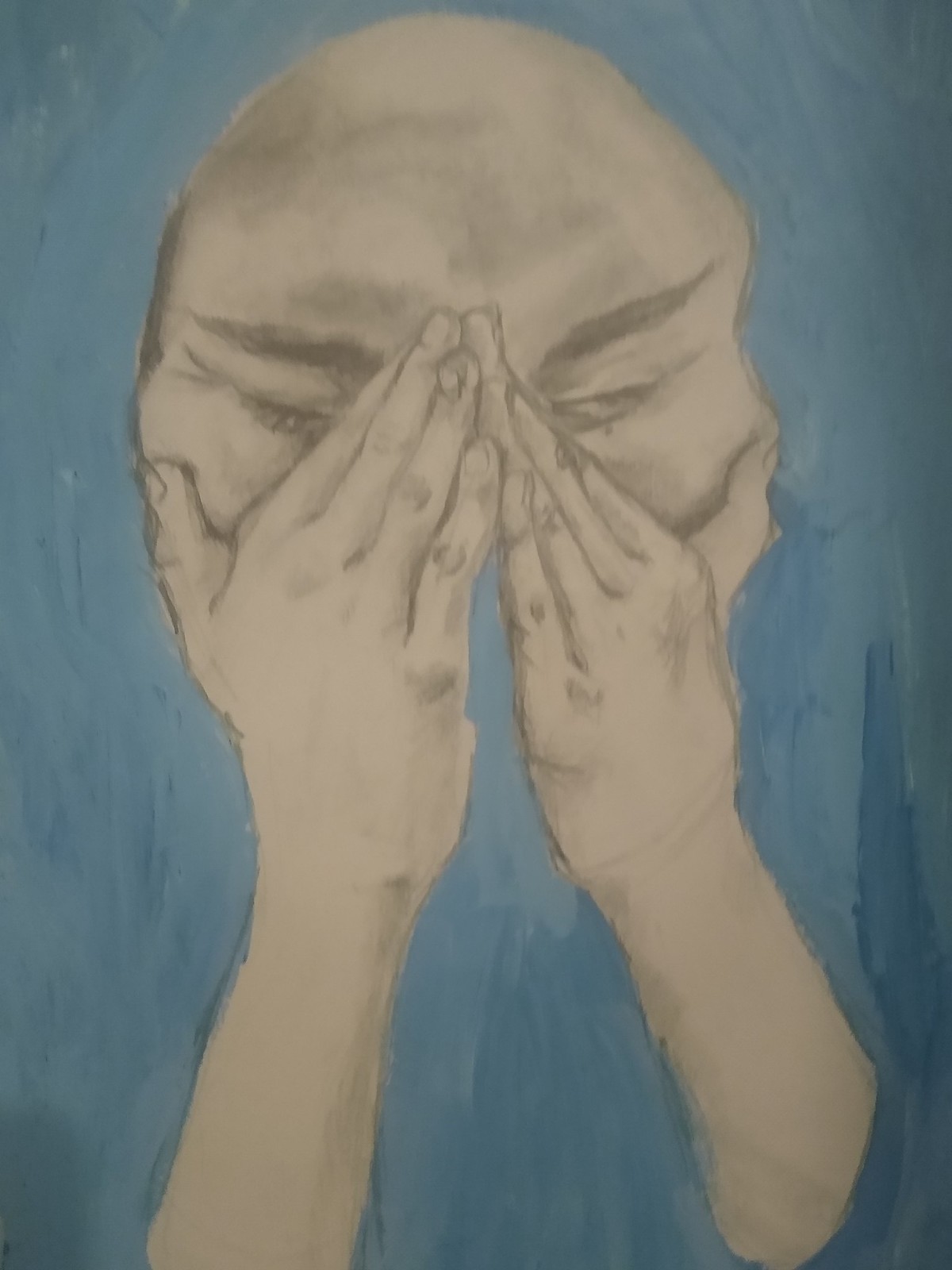A captivating artwork photograph showcases a meticulously detailed depiction of a person's face and hands. The subject's hands are brought together in a near-praying position, resting around the nose, creating an evocative expression of contemplation or introspection. Intriguingly, the lower half of the face, below the palms, is intentionally left out, adding an element of mystery to the piece. The background features a serene blue hue, painted with brushstrokes that contrast beautifully with the subject. The artist masterfully combines mediums, using both paint and blended pencil techniques. The face, characterized by a bald head and thick, defined eyebrows, along with the hands, is expertly shaded in pencil, showcasing intricate details and a realistic texture. This blend of styles and the enigmatic composition make the artwork a profound and thought-provoking visual experience.